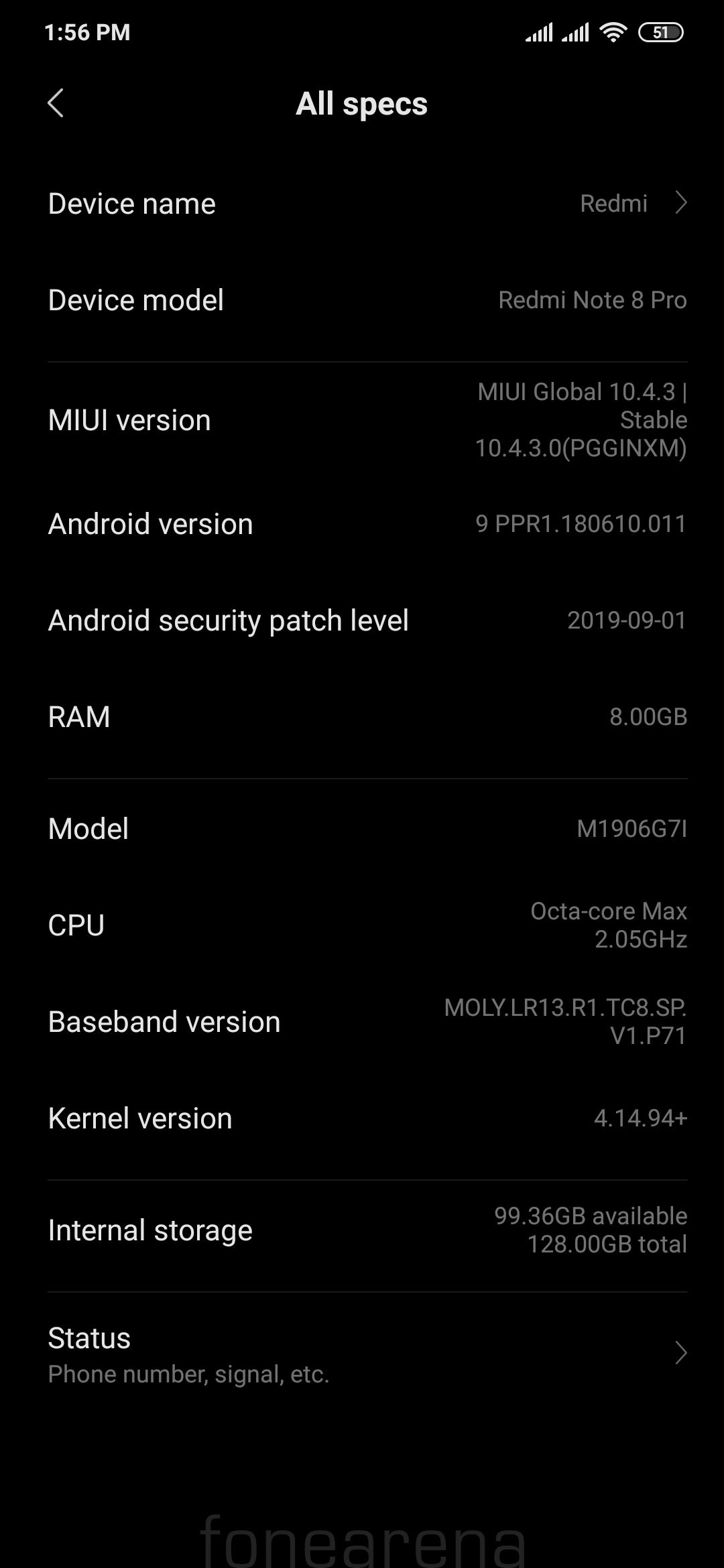The image is a vertical rectangular screenshot from a cell phone with a predominantly dark black background. 

At the very top, the white text displays the time as 1:56 PM. Below the time, centrally positioned, there's a bold white heading that reads "All Specs," accompanied by a small left arrow on the extreme left edge.

Below this heading, the content is organized into a vertical list of specs, all in bold white font. The categories listed are:
- Device Name
- Device Model
- MIUI Version
- Android Version
- Android Security Patch Level
- RAM Model
- CPU
- Baseband Version
- Kernel Version
- Internal Storage
- Status

Under "Status," in smaller white font, additional details such as "Phone Number," "Signal," etc., can be found.

Lower down, towards the bottom of the page, the grayed-out text reads "FO N E A R E N A," with spaced-out characters.

On the right side of the image, a column of text primarily consisting of numbers and technical details is visible. It begins with "REGMI" in uppercase letters, immediately followed by a small right arrow. Below this, "Redmi Note 8 Pro" is specified. Following this are various technical details and numerical data relevant to the device's specifications.